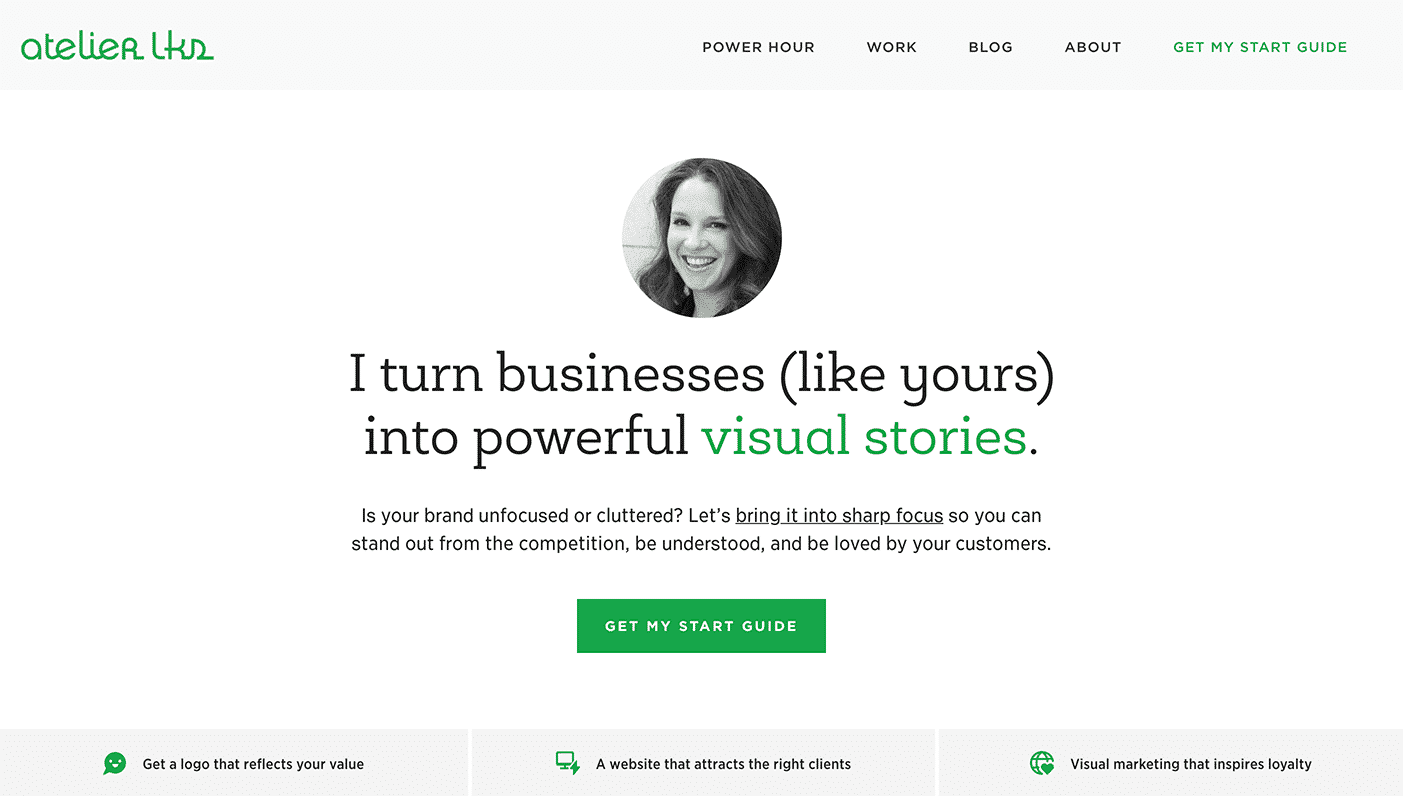This screenshot captures a segment of a website builder app, specifically highlighting the visual identity of 'Atelier OKS'. At the top of the page, 'Atelier OKS' is prominently displayed. Adjacent to this, a navigation menu features categories such as Power Hour, Work, Blog, About, and Get My Start Guide, with the latter option distinctly marked in small green letters.

Dominating the main body of the webpage is a clean white background. Centrally placed is a small, circular profile picture of a woman. Directly beneath her photo, a bold statement reads, "I turn businesses like yours into powerful visual stories," with the phrase "like yours" enclosed in parentheses and "visual stories" highlighted in green font.

Below this main statement, a centered, smaller black text poses the question, "Is your brand unfocused or cluttered?" It follows up with, "Let's bring it into sharp focus so you can stand out from the competition, be understood, and be loved by your customers." This call-to-action is followed by a prominent green button labeled "Get My Start Guide".

At the bottom of the screenshot lies a gray footer bar incorporating key service highlights paired with relevant icons: a chat bubble icon linked with "Get a logo that reflects your value", a laptop icon next to "A website that attracts the right clients", and a globe icon associated with "Visual marketing that inspires loyalty".